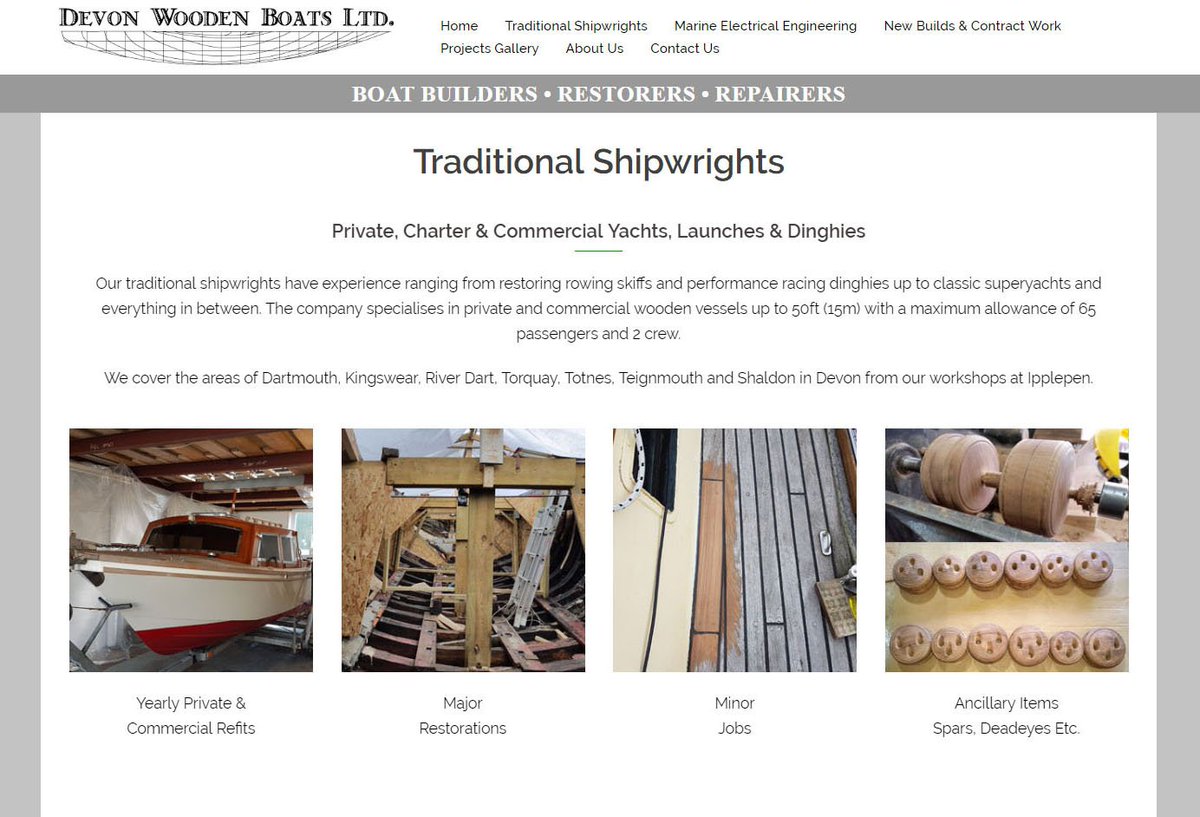The advertisement for Devon Wooden Boats Limited showcases their services as traditional shipwrights, marine electrical engineers, and new boat builders. The ad is set on a white background framed by a thick gray border on all sides except the bottom. The upper left-hand corner features the company's name, "Devon Wooden Boats Limited," along with their logo, which depicts the structure of a boat. Adjacent to this are clickable tabs labeled Home, Traditional Shipwrights, Marine Electrical Engineering, New Builds and Contract Work, Projects Gallery, About Us, and Contact Us.

Prominently titled "Traditional Shipwrights," the ad's central feature includes the text, "Private, Charter, and Commercial Yachts, Launches, and Dinghies." Below this title is a detailed paragraph explaining their services. At the very top of the gray border, large white text separated by dots reads, "Boat Builders • Restorers • Repairers."

The bottom section of the ad displays four aligned photographs, each with a descriptive label. The first photo on the left, under "Yearly Private and Commercial Refits," shows a red and white boat. Next to it, under "Major Restorations," is an image of a boat's infrastructure undergoing repair. The third photo, titled "Minor Jobs," depicts refinished teak boards being painted brown. The final image on the right, labeled "Ancillary Items, Spars, Deadeyes, etc.," shows various boat parts, including a wooden dumbbell and round wooden discs with cutouts.

In summary, this detailed advertisement effectively highlights Devon Wooden Boats Limited's expertise and range of services through concise text and illustrative images.